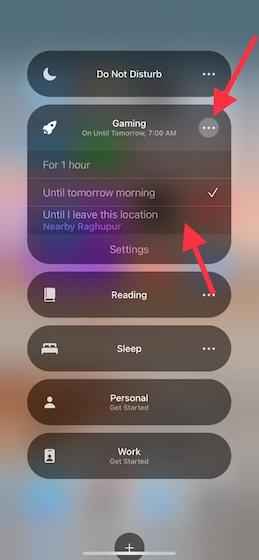The image is a screenshot of a mobile device's "Do Not Disturb" settings. At the top of the screen, "Do Not Disturb" is displayed in white font, accompanied by a half-moon icon on the left and three vertical dots on the right. Below this, there is a notification related to a gaming schedule which reads, "Gaming on until tomorrow 7 AM," again with the three dots to the right. A red arrow points to these dots. 

Further down, there is an option that says "For one hour," and another that reads "Until tomorrow morning," with a checkbox next to it. Under that, the setting reads "Until I leave this location," listed under the section marked "Nearby." The name "Ray Cooper" appears adjacent, with another red arrow pointing upwards towards the previous text.

Below this, the text "Settings" is displayed. Underneath it, there is a white font label "Reading," with a small picture of a book to the left and three dots to the right. Directly below, an image of a bed appears with the label "Sleep," followed by the three dots. Underneath, the sections "Personal" and "Get started," and "Work" and "Get started" are displayed sequentially.

This detailed overview describes the different options and icons presented in the "Do Not Disturb" settings of the screenshot, along with visual indicators such as red arrows pointing towards relevant elements.